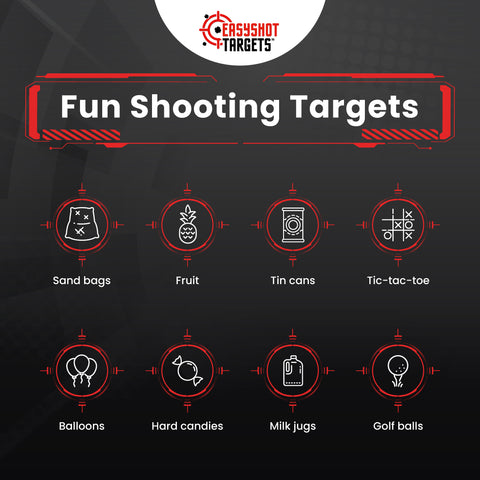The image features a dark gray square with prominent red and white text and graphics. At the very top, there's a distinct white semicircle containing a red and black logo that reads "Easy Shot Targets," featuring a red bullseye in the upper left corner. Below this, centrally placed, is the bold white text "Fun Shooting Targets," enclosed in a red rectangular border. The bulk of the image showcases two rows, each containing four target icons, depicted as red circles with white graphics inside.

The top row starts with:
1. Sandbags – illustrated by a graphic of a sandbag.
2. Fruit – represented by a pineapple image.
3. Tin Cans – shown as a can with a bullet hole.
4. Tic Tac Toe – depicted as a Tic Tac Toe game board.

The bottom row displays:
1. Balloons – illustrated by three balloon graphics.
2. Hard Candies – represented by a wrapped candy.
3. Milk Jugs – depicted as a plastic gallon jug.
4. Golf Balls – shown as a golf ball on a tee.

Each graphic corresponds to a label beneath it, providing fun and creative ideas for shooting practice targets that likely burst or shatter upon impact.